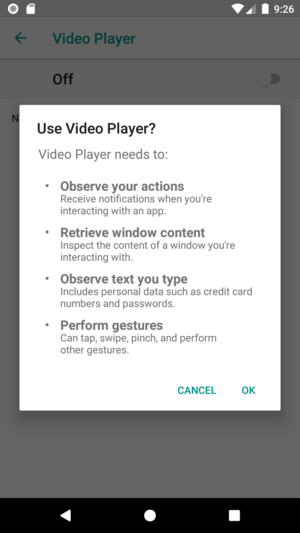This screenshot captures a cell phone screen, featuring a blend of status icons and a prominent permission request from a video player application. 

At the top of the screen, the status bar displays several icons. On the left side, there are a few unfamiliar symbols, while on the right, there is a Wi-Fi signal icon, a cell phone signal icon showing approximately half coverage, a battery status icon indicating a full charge, and the current time (9:26).

At the bottom of the screen, a black navigation bar includes three icons: a back button on the left, a circular home button in the center, and a square symbol representing recent apps on the right.

The slightly grayed-out background shows faint text indicating "Video Player" and the word "off." However, the main focus of the screenshot is a prominent white pop-up box asking for permissions. The pop-up reads: "Use Video Player?" and lists the following permissions the app requires:

- **Observe your actions:** Receive notifications when you're interacting with an app.
- **Retrieve window content:** Inspect the content of a window you're interacting with.
- **Observe text you type:** Includes personal data such as credit card numbers and passwords.
- **Perform gestures:** Can tap, swipe, pinch, and perform other gestures.

At the bottom of this pop-up box, there are two options labeled "Cancel" and "OK," allowing the user to either deny or accept these permissions before proceeding with the video player application.